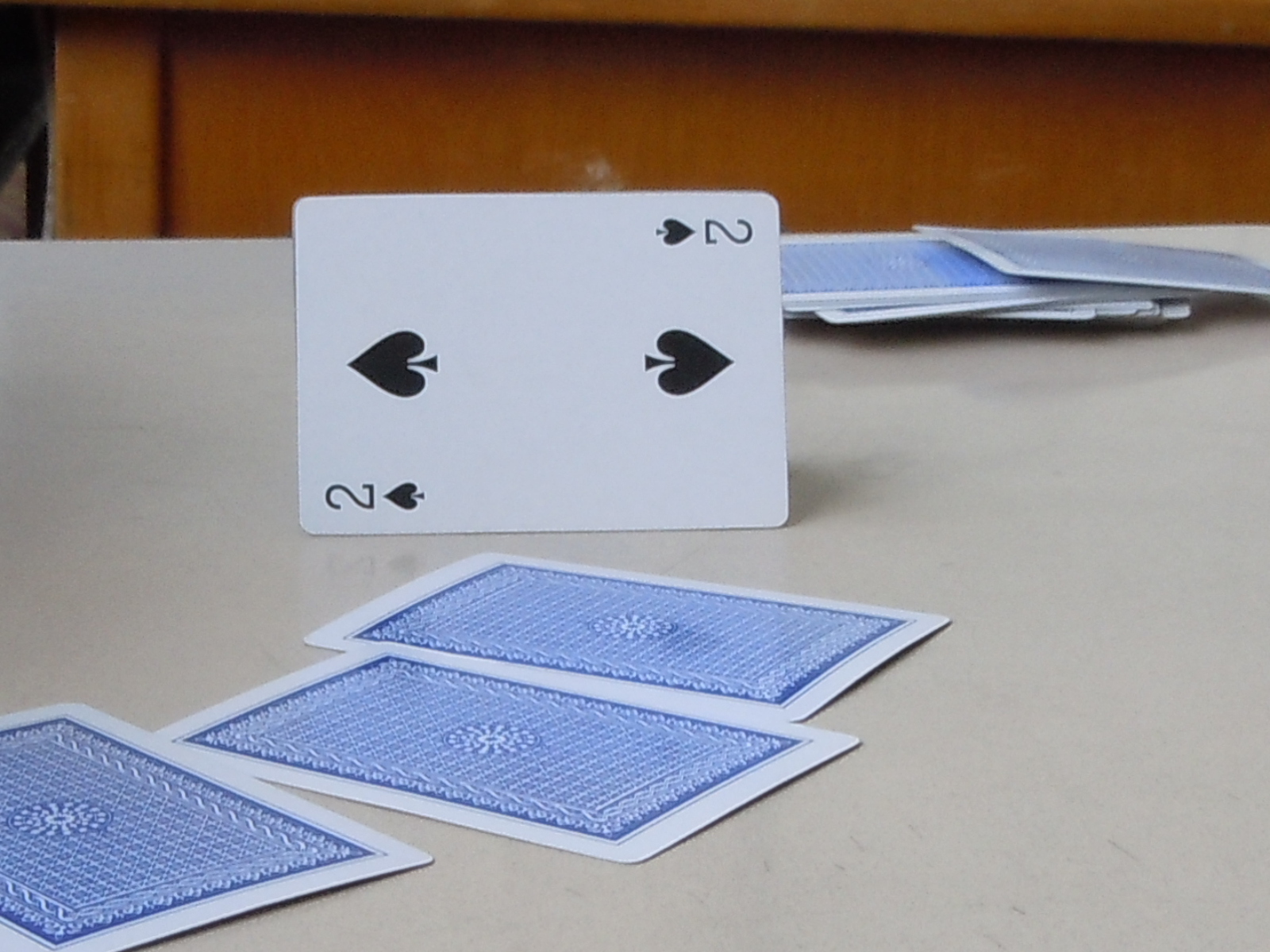This photograph captures a scene of playing cards laid out on a slightly reflective tabletop, possibly made of gray Formica, given the faint reflections. The playing cards feature blue backs adorned with an intricate geometric pattern that includes a central rosette, a grid structure, and ornate borders. In the center of the image, a Two of Spades card stands on its edge, facing the viewer mysteriously. In the foreground, three more cards lie face down in front of the upright Two of Spades. Behind these, an uneven, somewhat disorganized stack of additional cards can be seen, hinting at the tail end of a game or a hastily abandoned session. The background reveals the edge of the table or desk, adding depth and context to the scene, though it remains uncertain if a full deck is present due to the chaotic nature of the stack. The overall composition evokes curiosity about the circumstances leading to this arrangement, especially the precarious positioning of the Two of Spades card.